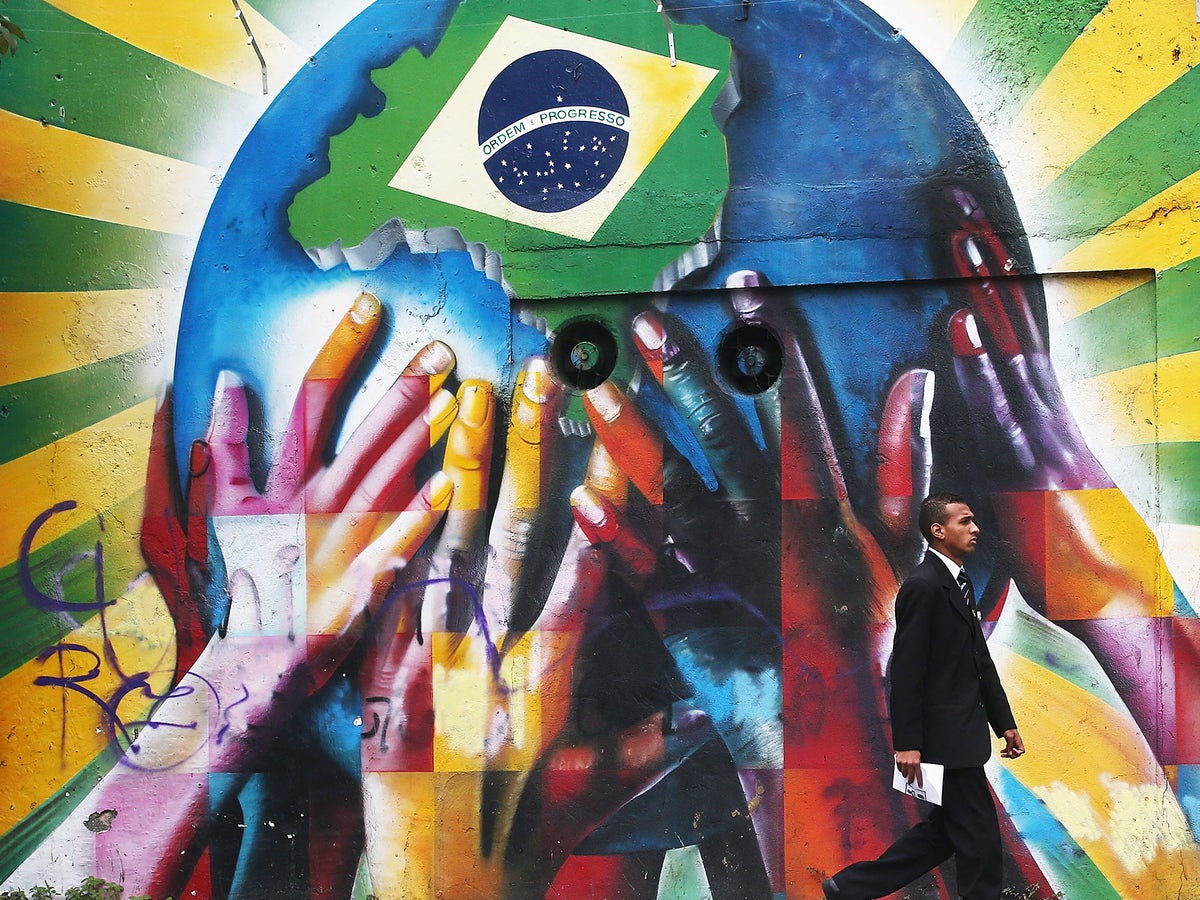The image captures a focused African-American man with short, almost shaved black hair, striding purposefully to the right side of the frame. He is dressed in a black business suit, complete with a dark-colored tie and a white undershirt, and he holds a piece of paper in his right hand. The man walks in front of a vivid mural painted on a large concrete building wall. The mural depicts a giant blue and green globe, suggesting the Earth, embraced by hands of various colors, including blue, orange, yellow, red, and more. These hands symbolize unity and diversity, collectively supporting the planet. Overlayed on the mural are striking green and yellow lines emanating from the globe. Prominently within the globe is the Brazilian flag, featuring a blue circle with a white band inscribed with "Ordem e Progresso," set against a green background. The scene is well-lit, adding to the clarity and vibrancy of both the man and the mural, which additionally includes some colorful graffiti elements.